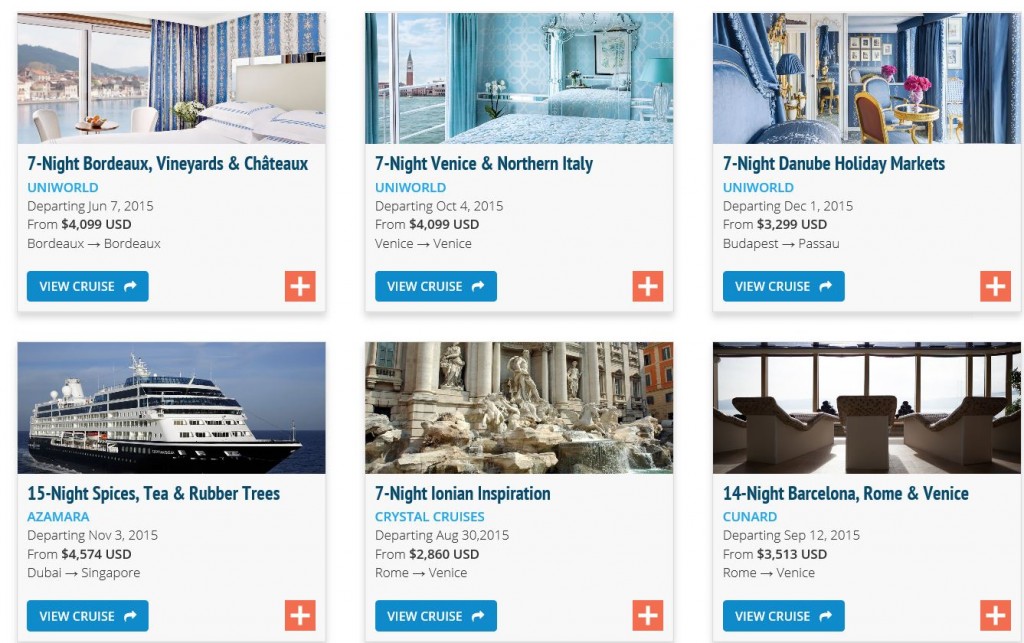Screenshot showcasing various cruise options:

Top Row:
1. **Seven Night Porto Vineyards and Chateau (Uniworld)**
   - **Departure Date:** June 7, 2015
   - **Price:** From $4,099 USD
   - **Route:** Bordeaux to Bordeaux
   - **Call-to-Action:** Blue "View Cruise" button

2. **Seven Night Venice and Northern Italy (Uniworld)**
   - **Departure Date:** October 4, 2015
   - **Price:** From $4,099 USD
   - **Route:** Venice to Venice
   - **Call-to-Action:** Blue "View Cruise" button

3. **Seven Night Danube Holiday Markets (Uniworld)**
   - **Departure Date:** December 1, 2015
   - **Price:** From $3,299 USD
   - **Route:** Budapest to Passau
   - **Call-to-Action:** Blue "View Cruise" button

Bottom Row:
1. **Fifteen Night Spices, Tea, and Rubber Trees (Azamara)**
   - **Departure Date:** November 3, 2015
   - **Price:** From $4,574 USD
   - **Route:** Dubai to Singapore
   - **Call-to-Action:** Blue "View Cruise" button

2. **Seven Night Ionian Inspiration (Crystal Cruises)**
   - **Departure Date:** August 30, 2015
   - **Price:** From $2,860 USD
   - **Route:** Rome to Venice
   - **Call-to-Action:** Blue "View Cruise" button

3. **Fourteen Night Barcelona, Rome, and Venice (Cunard)**
   - **Departure Date:** September 12, 2015
   - **Price:** From $3,513 USD
   - **Route:** Rome to Venice
   - **Call-to-Action:** Blue "View Cruise" button

Each cruise option is displayed within its own panel, featuring:
- A detailed itinerary
- A "View Cruise" button in the bottom left corner
- An orange square with a plus sign in the bottom right corner
- A snapshot of the room you'll be staying in.